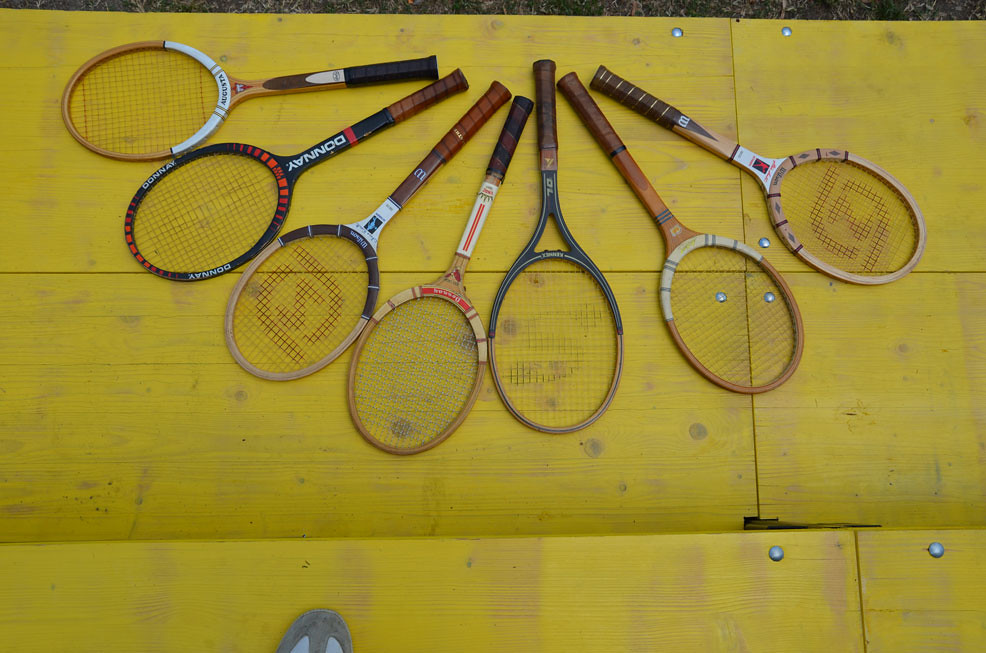The photograph features seven vintage wooden tennis rackets, each with leather-wrapped handles, arranged in a semi-circle on a yellow wooden surface. The rackets are lying face down, revealing a variety of colored frames, including shades of navy blue, light blue, and white, with some featuring purple and white accents. The surface beneath them is visibly worn and dirty, showcasing bolted sections that retain the wood grain texture. In the foreground on the lower right, a portion of the photographer's tennis shoe is visible. The strings of the rackets are made from nylon thread, and some of the racquets have visible branding with the letter 'S' on the netting.